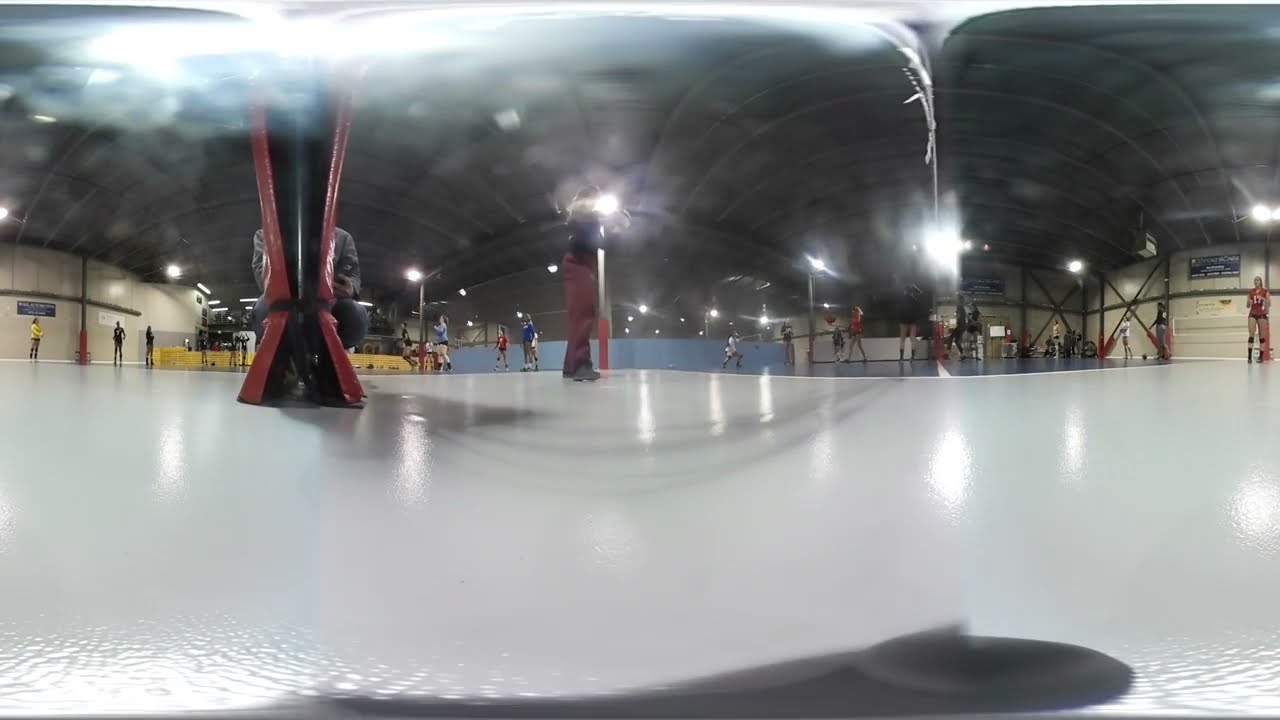This panoramic photograph depicts an indoor skating rink under a distinctive black roof adorned with white lights, creating a somewhat distorted but expansive view of the scene. The gleaming, pure white ice stretches across the foreground, with several skaters visible in the distance, engaged in various activities. One skater, identifiable by a black long-sleeve shirt and brown pants with the number 7, appears to be in mid-motion, possibly practicing for a routine. On the left side, a skater is captured performing an acrobatic jump, her skates and head elevated well off the ice. To the right, a padded pole with red cushioning and a white wall are visible, extending towards a door that leads to a non-skating area. Above, the ceiling's black arches reflect the lights, adding to the rink’s striking ambiance. A blue wall provides a backdrop where more skaters can be seen, some seemingly standing still or gliding slowly, with one woman in a red jersey possibly acting as a coach. The overall impression is of a dynamic and bustling practice environment under the artificial light of the indoor rink.